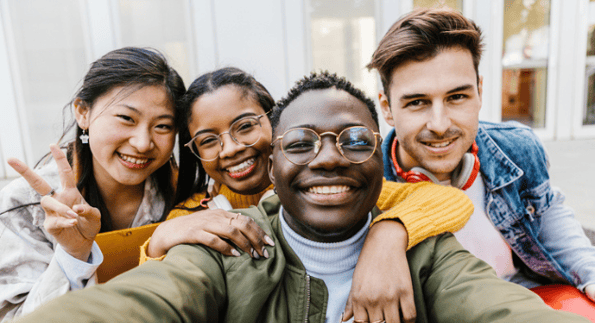A joyful selfie captures a group of four friends against the backdrop of a white building with long, narrow windows. The central figure—a smiling African American man with gold-rimmed glasses, a white turtleneck, and a green jacket—extends his arm to take the picture. To his left is a young Asian woman with black hair, adorned in a white coat and earrings, flashing a peace sign. On his right, a brown-skinned woman with glasses and black hair beams brightly in a yellow ribbed sweater, her arm draped lovingly around him. Completing the group is a Caucasian man with short brown hair and stubble, sporting a denim jacket over a white shirt, red headphones around his neck, and red pants. Despite the background being blurred, the friends' radiant smiles and camaraderie shine through vividly.